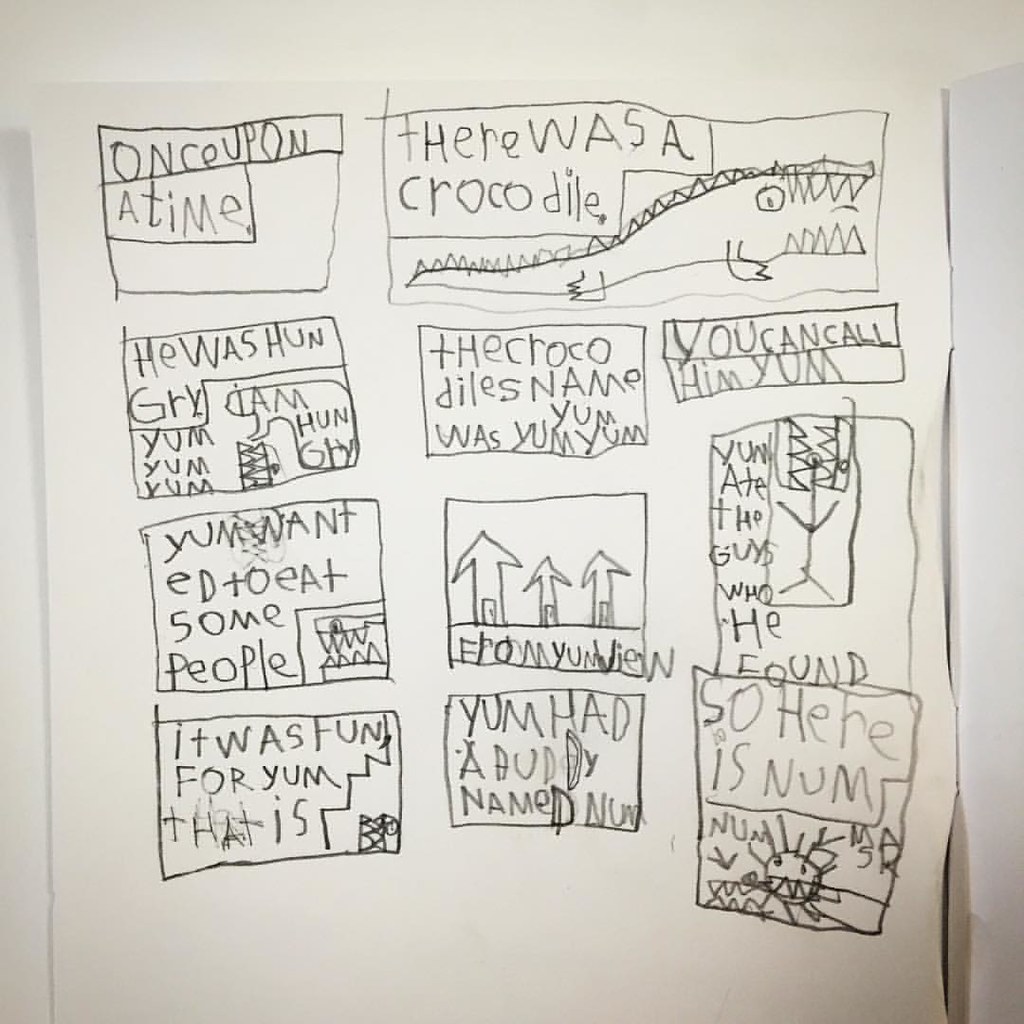The image depicts a black-and-white photograph of a large, white storyboard page, drawn and written by a young child in juvenile handwriting. The storyboard is presented in a square format and consists of 11 individual boxes distributed over four lines, each containing hand-drawn images and text. 

In the upper left corner, the first box reads, "Once upon a time." To the right, the next box introduces, "There was a crocodile," accompanied by a pencil drawing of a crocodile with prominent large teeth, an eye, and detailed scales on its back. Further along, the text continues with, "He was hungry," and a speech bubble declaring, "I am hungry. Yum, yum, yum." The next box reveals the crocodile's name, "Yum, Yum, Yum," and suggests, "You can call him Yum."

The story progresses to show Yum expressing his desire to eat people and humorously recounts how Yum ate the people he found. Additionally, the storyboard introduces another character named Num, illustrated in the final box on the bottom right with the caption, "So here is Num."

The entire storyboard is drawn in a comic book style, all in black and white, showcasing the child's creative narrative and artistic expression.